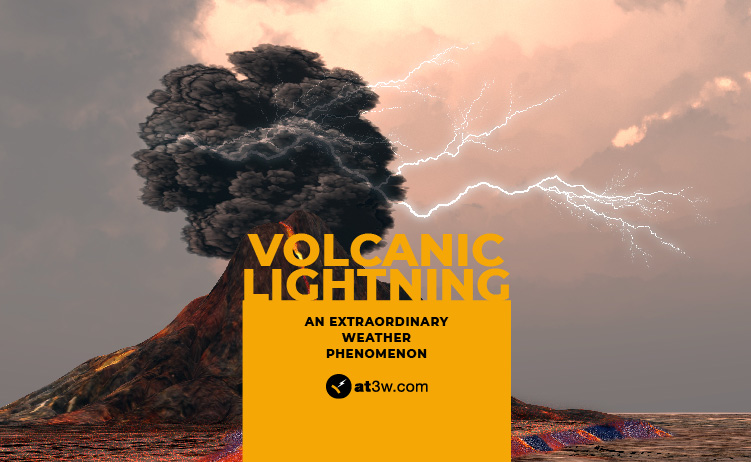The image is a dynamic and vibrant color photograph, prominently featuring an erupting volcano. Thick black plumes of ash and smoke billow skyward, resembling a mushroom cloud, while vivid streaks of volcanic lightning arc across the right side of the scene. Lava streams can be seen cascading down the volcano's slopes, adding to the dramatic spectacle. Behind the volcano, additional peaks are visible, suggesting a mountainous, likely volcanic, landscape. The sky is a mix of dark grays and brighter hues towards the horizon, hinting at the sun peeking through the clouds. The photograph is overlaid with a saturated yellow text box at the bottom center. It reads “Volcanic Lightning: An Extraordinary Weather Phenomenon,” with the logo “AT3W.com” included, indicating this is likely an advertisement or promotion for a website with further information about this natural occurrence.